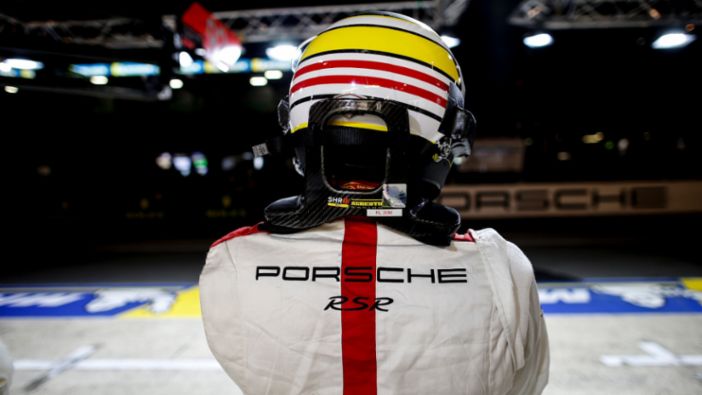The image depicts a realistic photograph of a race car driver from Team Porsche, captured in a horizontally oriented shot at night, either indoors or on an outdoor track with bright overhead lighting. The driver is seen from behind, standing amidst a raceway setting, which features prominent Porsche and Michelin signs. The person, whose gender is indeterminate due to their helmet obstructing their face, is clad in a white racing uniform with the Porsche RSR designation in black text and a red stripe down the middle. They are also wearing a distinctive yellow, white, and red helmet, secured with a black neck brace for support. The scene is slightly blurred in the background, possibly using a portrait setting in the camera, focusing intently on the driver who seems to be waiting either for their turn to race or having just completed a race. The ground shows some blue and yellow writing, enhancing the professional racing atmosphere. The environment, bustling with race-related gear and lighting, sets a vivid and immersive backdrop for this poised and focused race car driver.